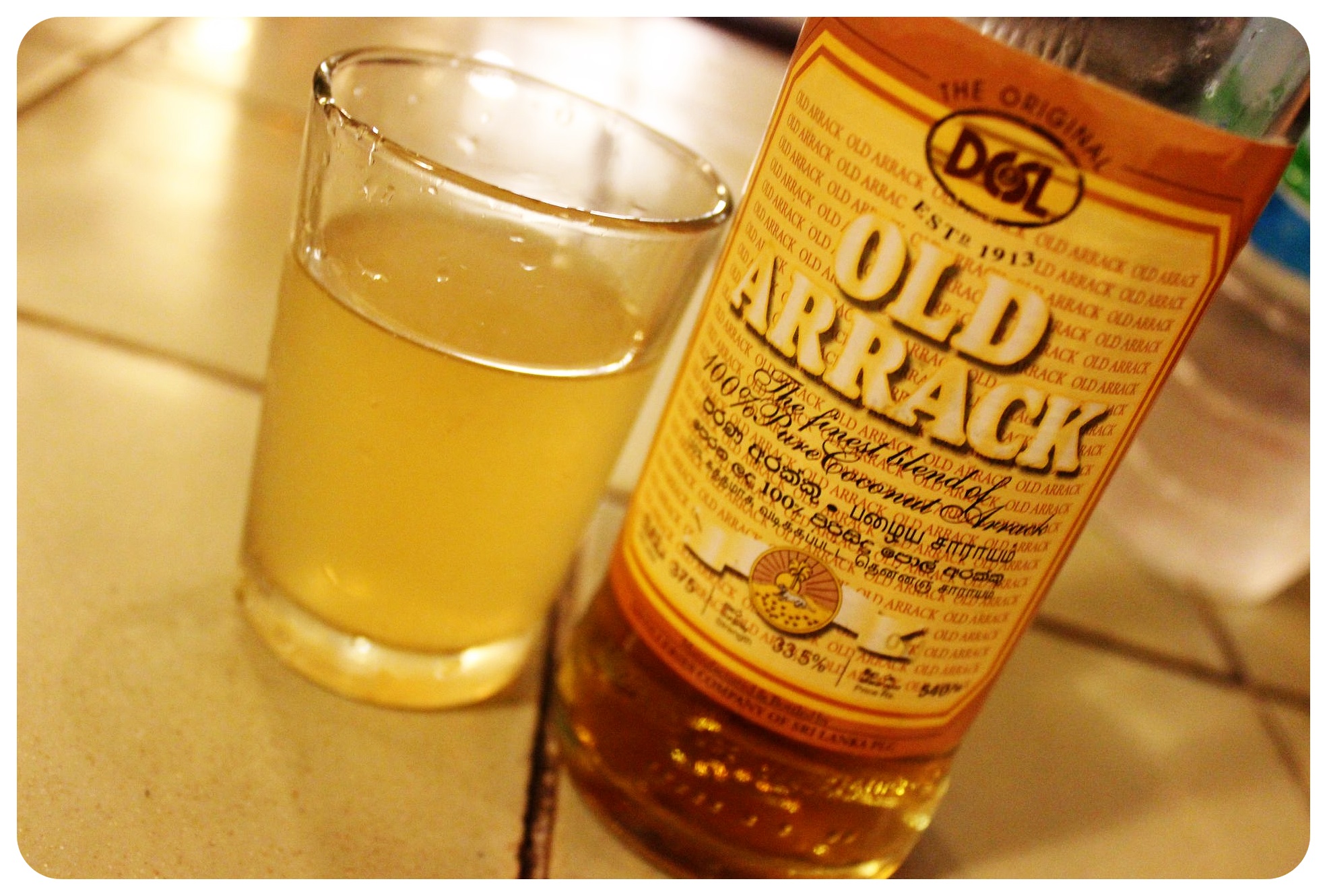The image depicts a diagonally angled scene featuring a bottle of Old Arrack and a glass filled with the same golden-amber liquid on a yellow tile countertop with brown grout lines. The bottle has an orange and yellow label with white lettering, reading: "The Original DNL, EST 1913, Old Arrack, The Finest Blend of 100% Pure Coconut," and a notation of "33.5% alcohol." There’s a logo at the bottom featuring a ribbon with a gold coin. In the background, a water bottle and several other objects are visible, adding context to the setting.